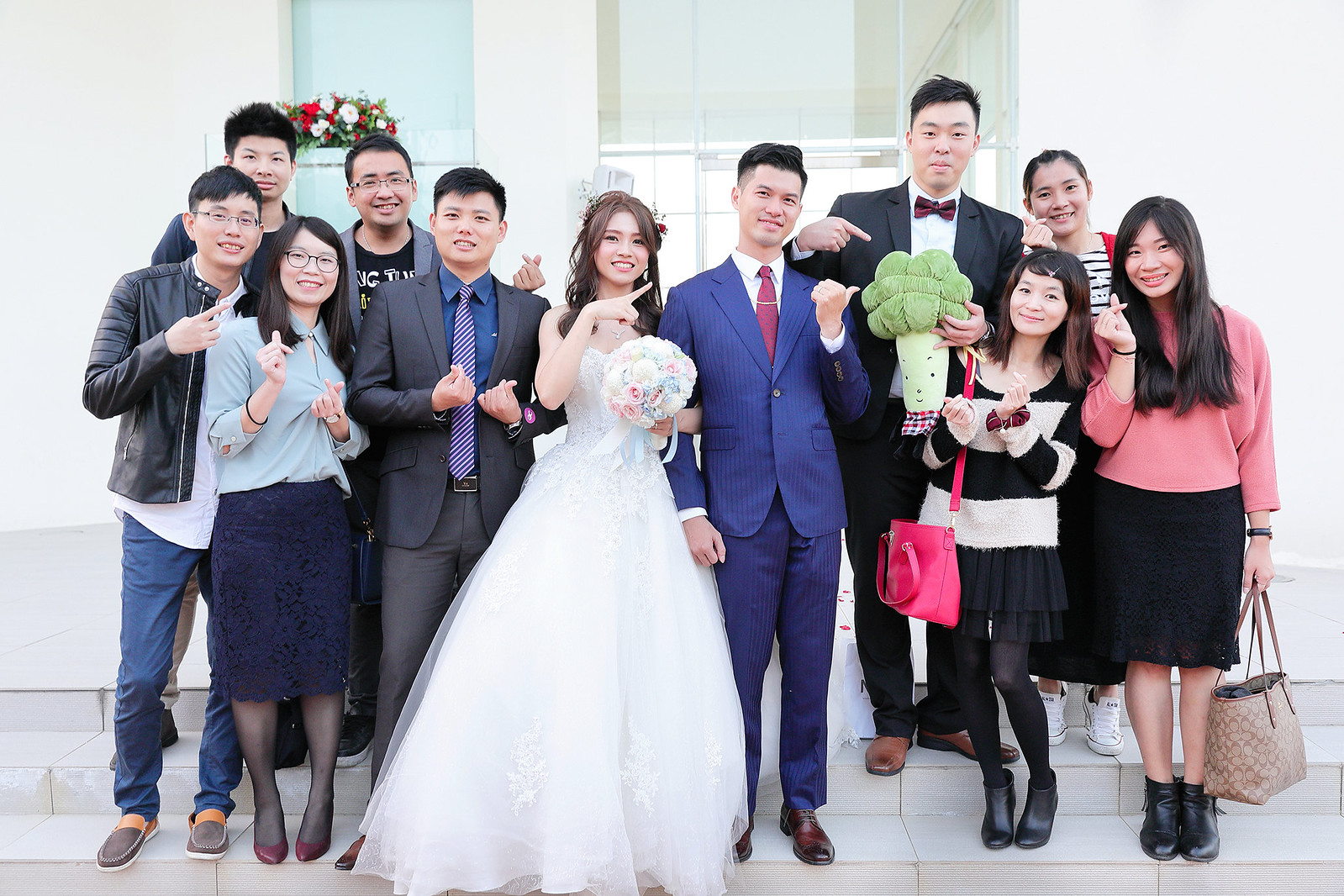This vibrant color photograph captures a joyous wedding celebration of an Asian couple surrounded by their family and friends. In the center, the bride, approximately 18 or 19 years old, stands elegantly in a strapless white gown with a long, floor-length skirt made of netting. She holds a bouquet of white and light pink flowers in her left hand, partially obscuring her bodice. Her long brown hair cascades just past her shoulders, possibly adorned with a subtle headpiece. To her right stands the groom, around 20 years old, in a well-fitted navy suit, brown leather shoes, and a red tie, with short black cropped hair.

The wedding party, consisting of about eight or nine people, positions themselves on white marble-effect stairs, their divisions marked by dark, narrow slits. The group is diverse in attire, with some men in suits or jeans and leather jackets, and women in blouses, skirts, and even a hot pink purse. Both the bride and groom, along with other members, are engaged in playful gestures: many point towards a distinctive plush toy held by the tallest man in the photo, a whimsical stuffed broccoli with a face and a plaid bib, while others form heart shapes with their fingers. This casual and joyful scene, with everyone smiling towards the camera, encapsulates the festive spirit of the occasion.